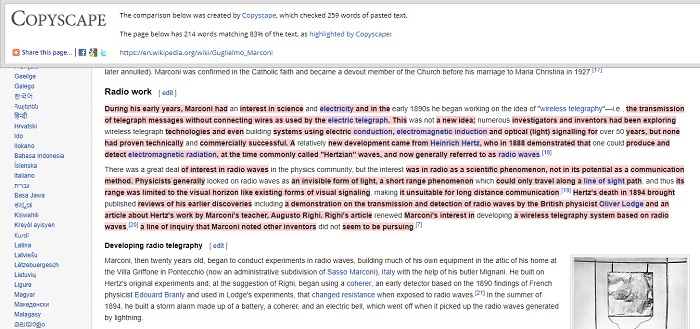**Detailed Caption:**

The screenshot features a page reviewed by Copyscape, a plagiarism detection tool highlighted in blue. The tool analyzed 259 words of the posted text. On the left side of the screen, there is an option to "Share This Page." Next to it, there is a radio button labeled "work" and an "Edit" button highlighted in blue. The content is partially highlighted in red to indicate similarities detected during the early years. An excerpt about Marconi discusses his interest in science and electricity, the latter also highlighted in blue. Around the early 1890s, Marconi began exploring the concept of wireless telegraphy, with "wireless telegraphy" highlighted in blue. The term is explained as the transmission of telegraph messages without connecting wires, distinguishing it from the electric telegraph, also highlighted in blue. Although this concept was not new, with numerous investigators and inventors already exploring wireless telegraph technologies and building systems using electric conduction, as indicated by the transition between highlighted and non-highlighted text.